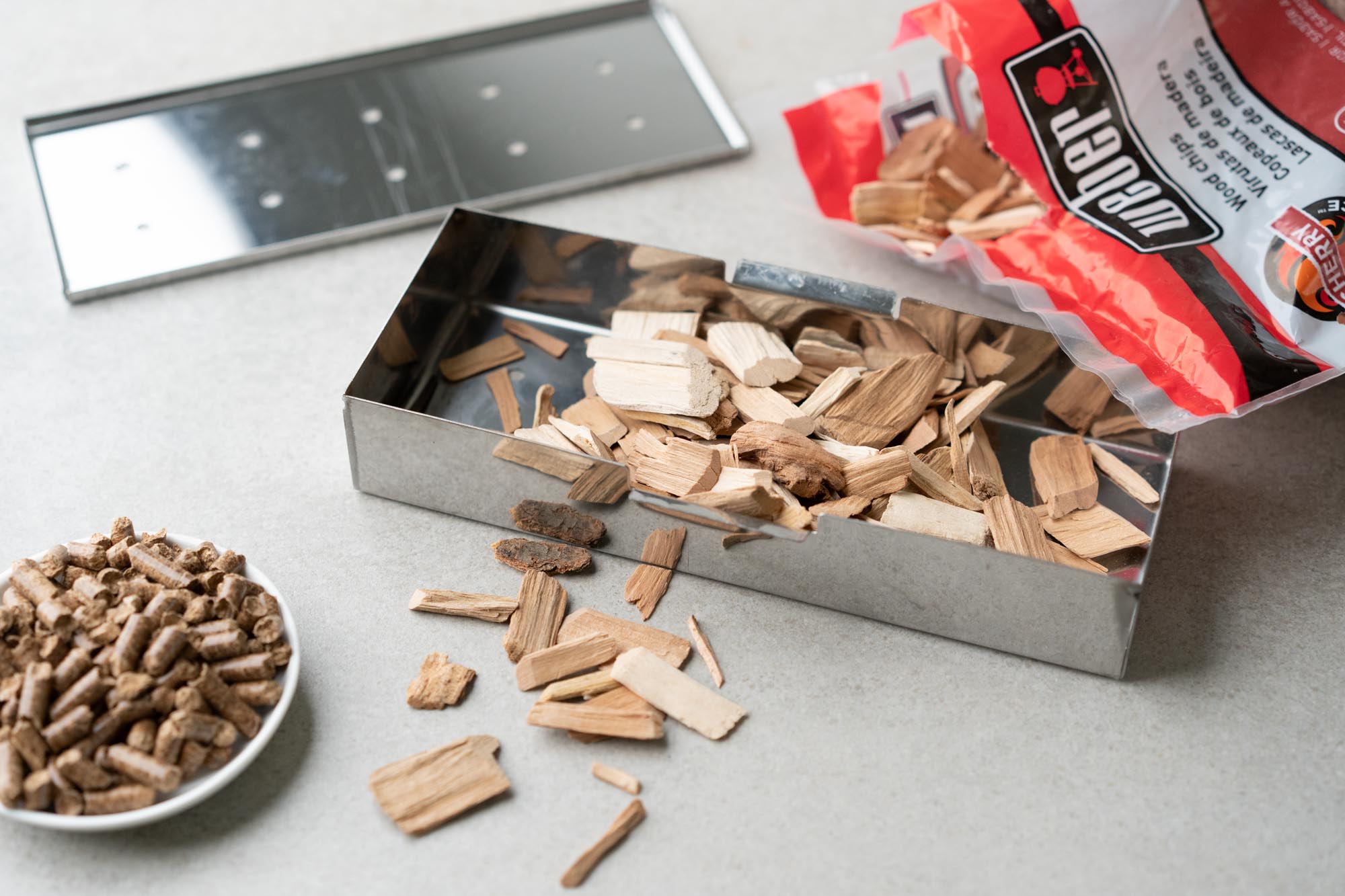The photograph displays a detailed grilling setup with various accessories meticulously arranged on a textured gray table. In the background, a diagonally positioned striped red, black, and white bag prominently labeled "Weber" in black text that reads "wood chips" in multiple languages. The word "Cherry" appears within a black and orange logo on the left side of the bag. Centered in the frame, a shiny, reflective, rectangular tin box, measuring approximately three inches by one inch, is filled with white and light brown wood chips, suggesting hickory due to the adjacent Weber bag. This metal container has a separate lid with ten evenly spaced holes, reminiscent of a domino, placed slightly blurred in the background to the left. Scatterings of wood chips are noticeable around the bottom of the tin box, also reflected on its polished surface. On the left, a small white dish holds a pile of compressed cylindrical wood pellets, raising curiosity about their exact purpose, potentially for fire aid or otherwise. The harmonious arrangement of these elements on the table forms a cohesive image emphasizing the essentials for a grilling session.